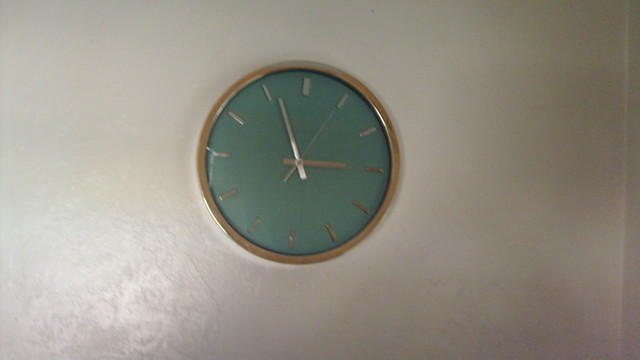The slightly out-of-focus photograph features a gray wall serving as the background. In the center of this wall hangs a clock with a gold-toned frame. The clock's face is a striking green, adorned with minimalist tick marks instead of traditional numbers, requiring the viewer to interpret the time using their familiarity with clock faces. The minute hand points to the 56-minute mark, the hour hand is close to 3 but not quite there, indicating the current time is 2:56. The second hand is precisely at the 5-second mark.